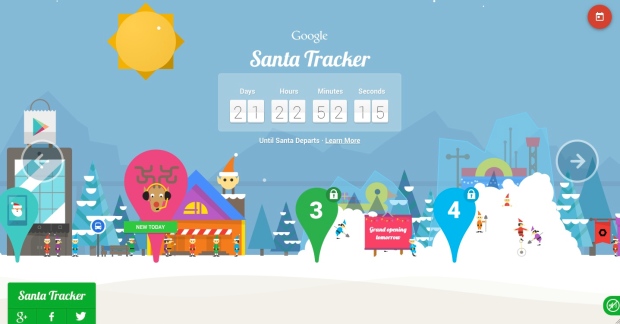The screenshot features the Google Santa Tracker interface, displaying a festive North Pole scene in anticipation of Christmas. The background is a serene pale blue, depicting a snowy landscape adorned with several elements. Central to the image is a cozy little house with a chimney, from which an elf cheerily pops out, adding to the holiday spirit.

Reindeers are seen mingling near the house, which is flanked by various buildings, including what appears to be Santa's iconic workshop. Numerous evergreen trees, heavily blanketed with snow, dot the landscape, with majestic mountains visible in the far distance. The scene is completed with a large snow pile where five or six elves are busily shoveling snow.

In the bottom left corner, a green rectangle with white text reads "Santa Tracker," accompanied by social media sharing options for Google+, Facebook, and Twitter. The top left corner of the image features a bright yellow sun, shining down on the snowy terrain. 

The bottom right corner has a green audio control tab, marked by a circled audio icon with a slash indicating mute. Flanking the image, both centrally on the left and right edges, are navigational arrows circled, likely to enable further exploration of the interactive scene. Snow is omnipresent, beautifully laying the groundwork for this enchanting digital portrayal of the North Pole.